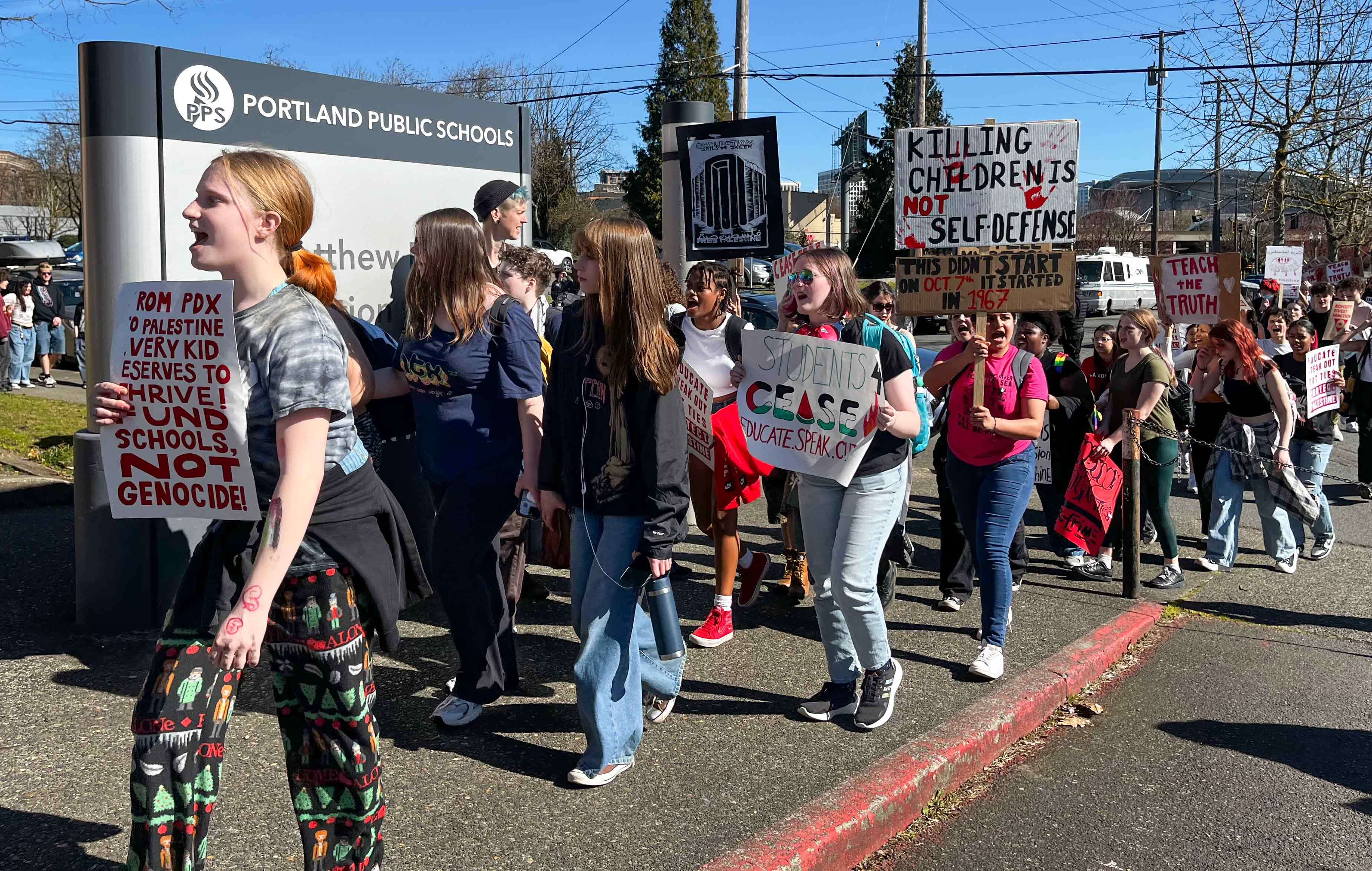The image depicts a high school student protest against the war between Israel and Palestine. The protest is taking place in front of a sign for Portland Public Schools, partially obscured by the students. It is a bright day in early spring, evident from the leafless trees and the students' attire, which includes both pants and short sleeves. In the foreground, a group of predominantly female students are marching, many holding handmade signs. 

The leading girl, identifiable by her red hair, holds a white sign with red letters reading, "10 million PDX to Palestine, every kid deserves to thrive, fund schools, not genocide," while she has hearts drawn on her hand. Another sign reads, "Killing children is not self-defense," with others stating, "Students cease education," "Every kid deserves to thrive," and "Teach the truth." 

The image also shows a larger background poster stating, "Killing children is not self-defense." Various students in the crowd, estimated to be around 30-40 strong, are visibly chanting and marching on the pavement. The diverse array of signs and the passionate expressions suggest a highly motivated and coordinated effort by the students to voice their concerns and demand action.